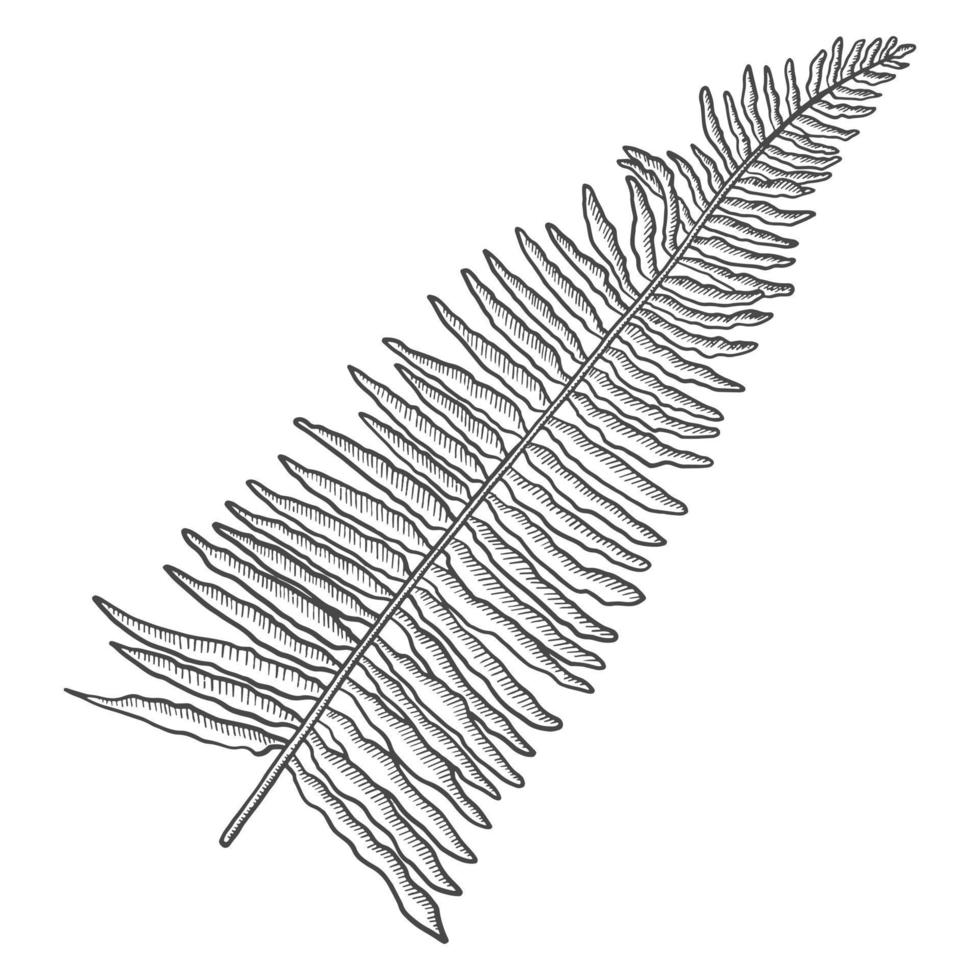This detailed black and white sketch illustrates a fern-like leaf against a white background. The drawing features a single elongated branch, diagonally oriented from the lower left to the upper right corner of the image at approximately a 50 to 60-degree angle. The center stalk, or stem, has a series of paired leaves emanating symmetrically from each side, starting at the bottom and getting progressively shorter towards the top. The leaves are elongated and tapered, with pointed ends that give the overall branch a triangular shape. The leaves are squiggly and lumpy in appearance, adding an organic texture to the otherwise simplistic design. At the very tip of the branch sits a solitary leaf, distinguished as the only one without a pair. The entire sketch stretches to the top of the image, emphasizing the tall and elegant nature of the leaf. There is no text within the image.